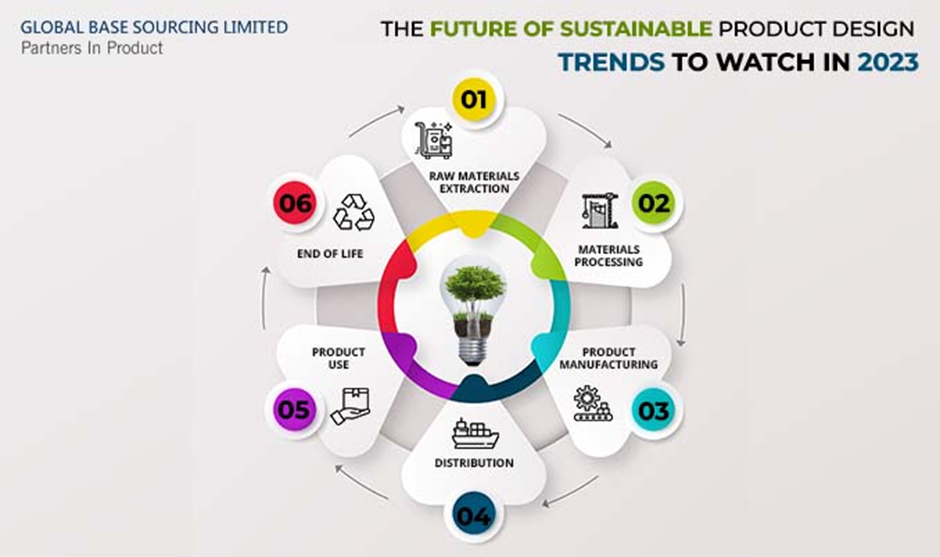The image is a detailed diagram set against a gray background, titled "The Future of Sustainable Product Design: Trends to Watch in 2023." At the top left, it reads "Global Based Sourcing Limited," followed by the subtitle "Partners in Product." The diagram, reminiscent of a fan or circle with heart or triangular-shaped segments, illustrates six interconnected stages of product lifecycle. Central to the circular design is an illustration of a lamp containing a tree, symbolizing sustainability and growth. 

Positioned clockwise around the lamp, each segment is labeled and color-coded to depict different stages: 

1. **Raw Materials Extraction** - Orange
2. **Materials Processing** - Green
3. **Product Manufacturing** - Aqua Blue
4. **Distribution** - Navy Blue
5. **Product Use** - Purple
6. **End of Life** - Red

Arrows guide the viewer through each stage in a clockwise manner, visually emphasizing the flow and interconnection between stages.